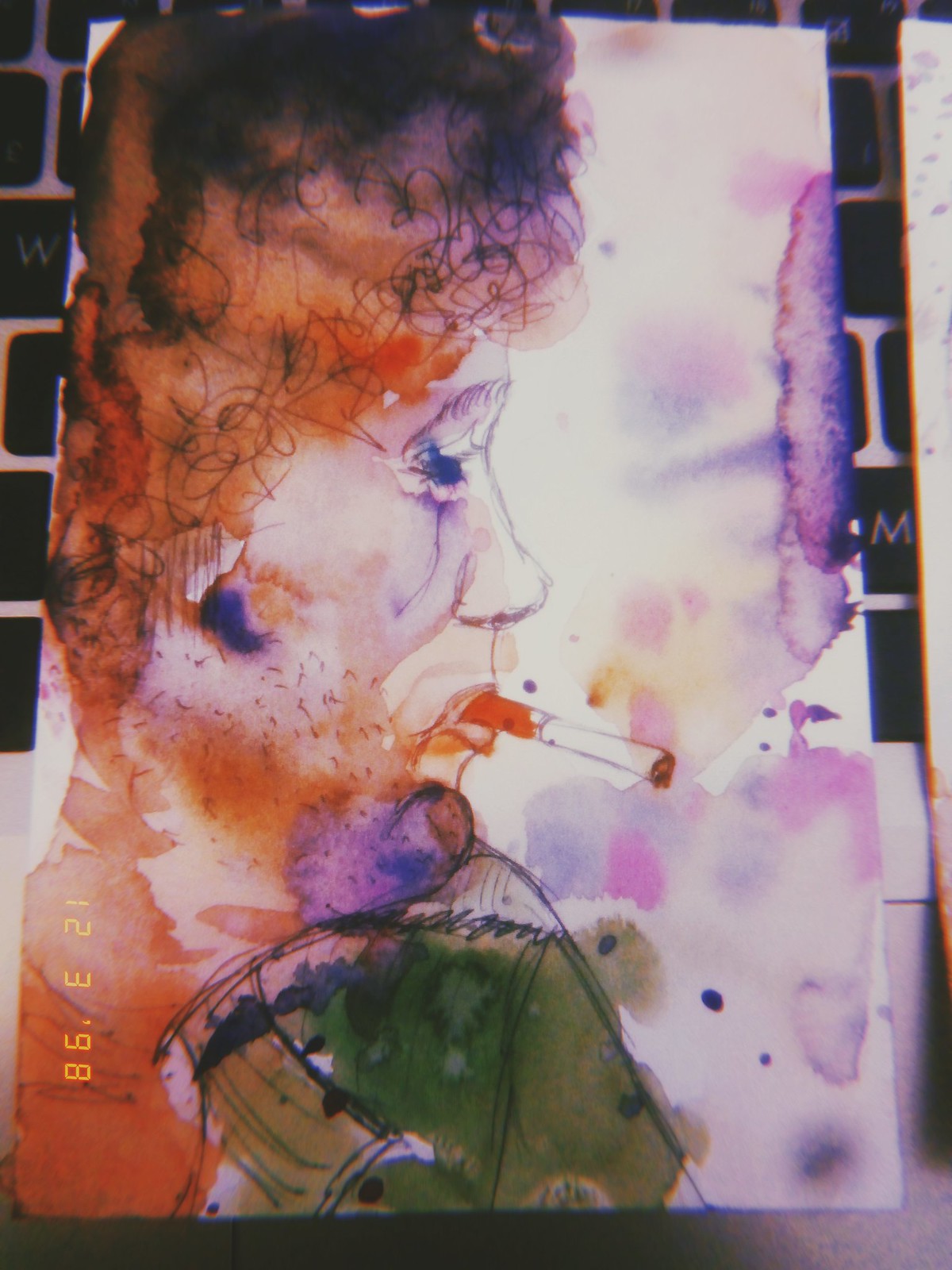The image depicts a watercolor painting on a white canvas, appearing as if it was created in an art class. The painting presents a side profile of an individual's face turned to the right, with a focus on the right eye, nose, and mouth. The person has highly detailed, curly hair in a mix of reds, oranges, browns, and black, and the hair reaches down to what might be an earring, marked by a blue area where the ear would be. The right eye has a blue iris, surrounded by white makeup and detailed eyebrows, although the makeup appears smudged, perhaps by water or rain. The person’s face has additional white markings typically associated with clown makeup, particularly around the eye and mouth areas. 

A cigarette with a red tip, seemingly lit, hangs from the mouth. The chin exhibits a blue hue interspersed with whisker-like lines. Below the chin, the person appears to wear a green top, although this area is somewhat unclear and blends into the background. The background itself is splattered with purples, yellows, and pinks, particularly smudged on the left-hand side, enhancing the impression of further water damage. Additionally, a digital number sequence, "12398," is visible to the side of the painting. The entirety of the piece seems to rest on a surface resembling black tile with white grout.